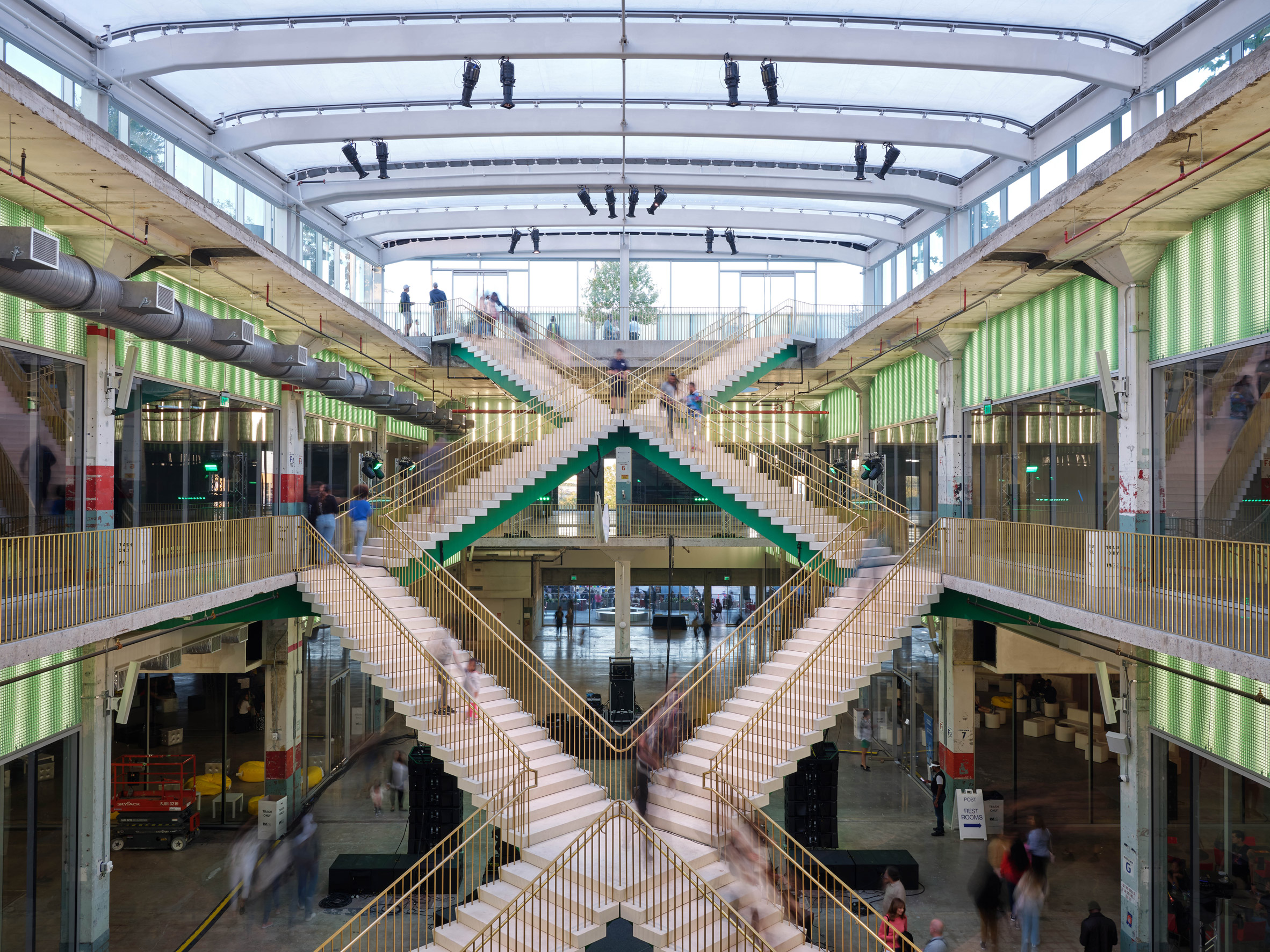This photograph captures a grand, ornately designed interior space that appears to be an empty, under-construction indoor mall spanning at least three stories. The focal point of the image is a set of cream-colored staircases, intricately designed, descending from both the left and right to create a striking "X" pattern in the center. These stairs feature elegant gold handrails, with the areas at the very top and bottom accentuated by dark green tones. The image is brightly illuminated by natural light streaming in through a mirrored and glass roof, suggesting it was taken during daylight hours.

The sides of the image showcase potential storefronts with large glass windows and vertical green and white striped awnings, but no discernible activity inside, reinforcing the sense of incompletion. There are scattered construction equipment and people visible at the lower level, though they appear blurry and are not the focus of the photograph. The ambiance is further characterized by the emptiness and vastness of the space, punctuated by occasional movement, likely captured in a time-lapse style, adding to the overall impression of an ongoing construction project.